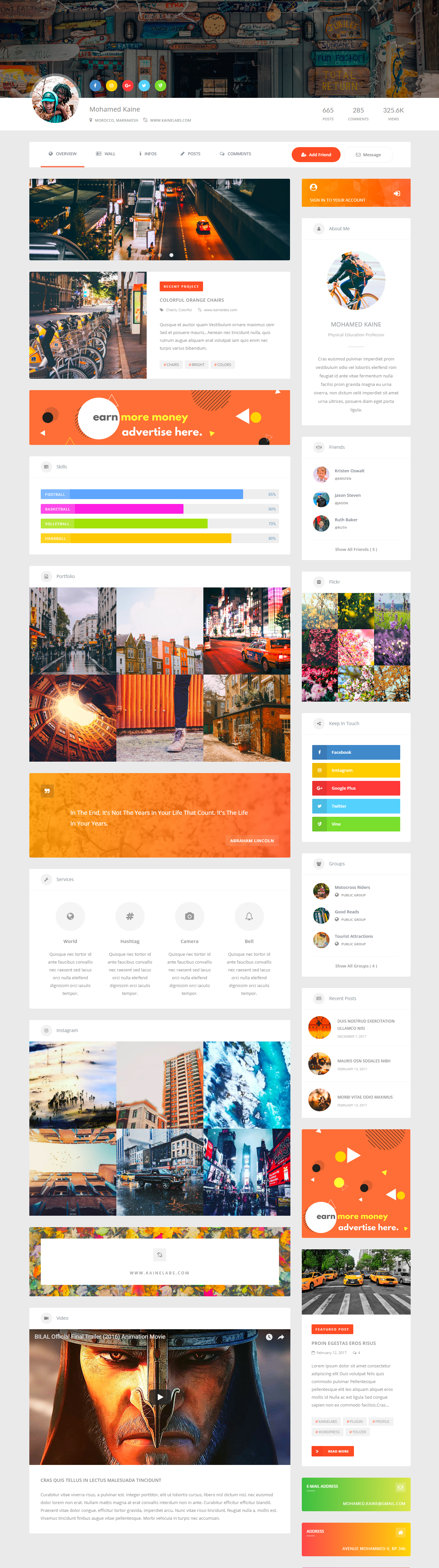This is a screenshot of a personal website belonging to Mohammed Kain, who is based in Marrakesh, Morocco. The website URL is www.kainelabs.com. The page appears to have been significantly resized to fit within a smaller view. The site boasts 665 posts, 285 comments, and 325,600 views. 

The content includes several city street photos featuring cars and bicycles. A recent project highlighted on the page involves vibrant, orange chairs, accompanied by descriptions in French, although specific translations are unclear. Various hashtags are associated with these images.

There is a section promoting advertisement opportunities with the message "Earn more money, advertise here." Additionally, there is a list of skills that includes football, basketball, volleyball, and a general mention of "ball."

At the bottom of the page, a quote reads: "In the end, it's not the years in your life that count, it's the life in your years." This website appears to be a personal blog or portfolio reflecting Mohammed Kain's projects, interests, and skills.